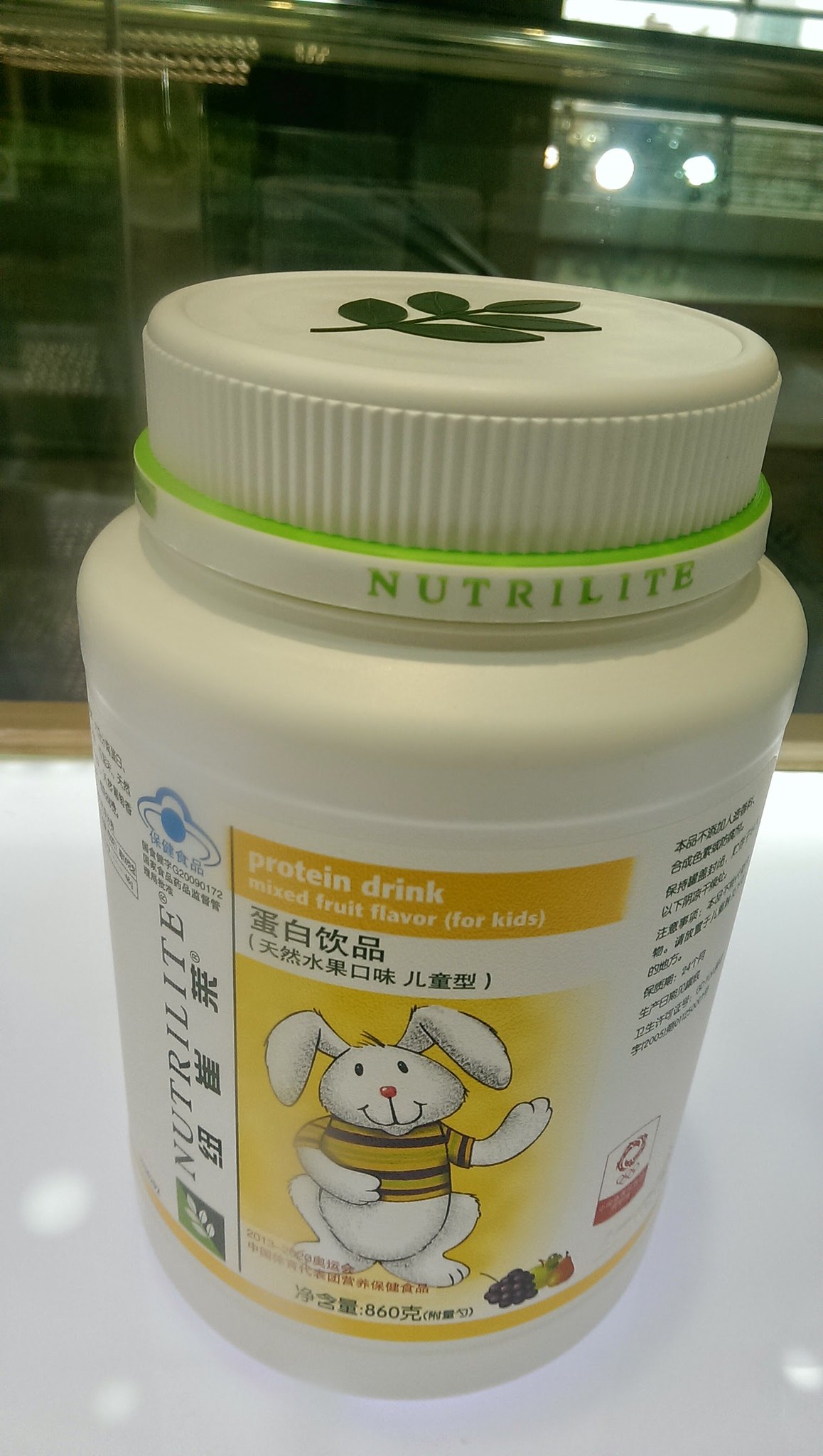This portrait-oriented photograph captures a white plastic jar prominently positioned in the frame. The jar features a green plant leaf placed atop its ribbed lid. Encircling the ribbed rim is a white band with a bright green top, marked with the brand name "Nutrilite" in bold green text. The jar's white label features a distinctive yellow section in the center, which reads "Protein Drink Mixed Fruit Flavor for Kids." Below this text, a charming cartoon illustration of a white rabbit dressed in a yellow, brown, and green t-shirt is depicted. Beneath the rabbit, vibrant renderings of fruits, including grapes, an apple, and a pear, add a colorful and playful touch to the label.